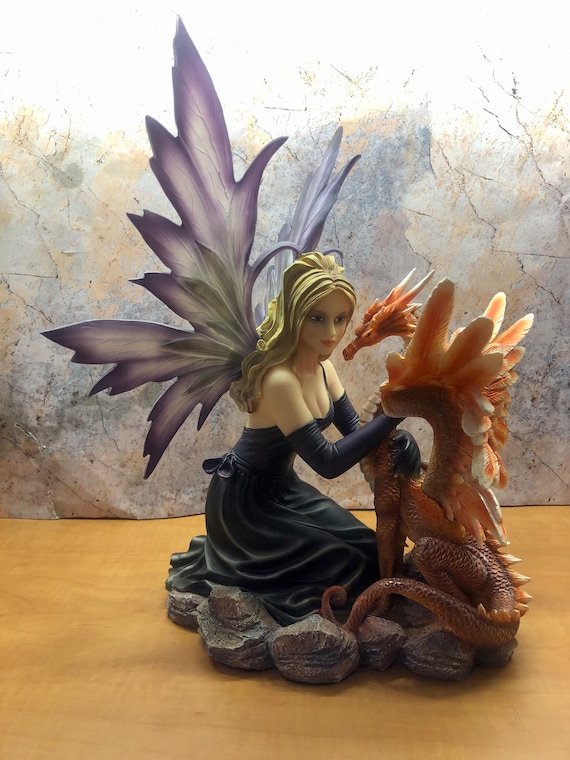A beautifully detailed statue depicting a graceful fairy in an intricately designed blue dress, adorned with delicate spaghetti straps. Her long, flowing blonde hair cascades gently over her shoulders, framing her serene expression. The fairy's impressive, large purple wings are fully extended, giving the impression they are poised to flap at any moment. She is kneeling down, tenderly holding and caressing a small dragon with vibrant orange and red scales, capturing a moment of intimate connection between the two magical creatures. The scene is rich with fantasy elements, bringing an enchanting fairy tale to life.